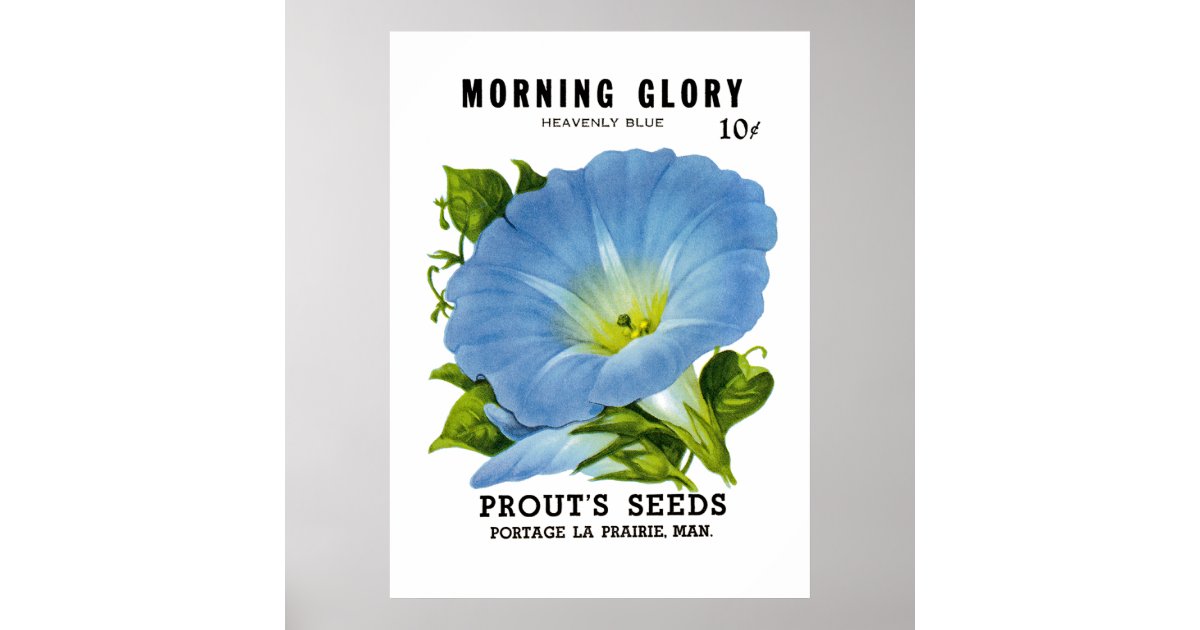This close-up product shot showcases a white packet of Morning Glory seeds, set against a light blue background. The packet features "Morning Glory" prominently in large black letters at the top, with "Heavenly Blue" written in smaller black font just below it. To the right of these, the price "Ten Cents" is also listed in black letters. Dominating the center of the packet is a watercolor illustration of a vibrant Morning Glory flower. This blue flower, with its delicate yellow center and accompanying green leaves, is detailed and lifelike, portraying open blossoms as well as budding flowers. Towards the bottom of the packet, "Prouts Seeds" is displayed in large black letters, followed by the location "Portage La Prairie, Manitoba" in smaller black text.